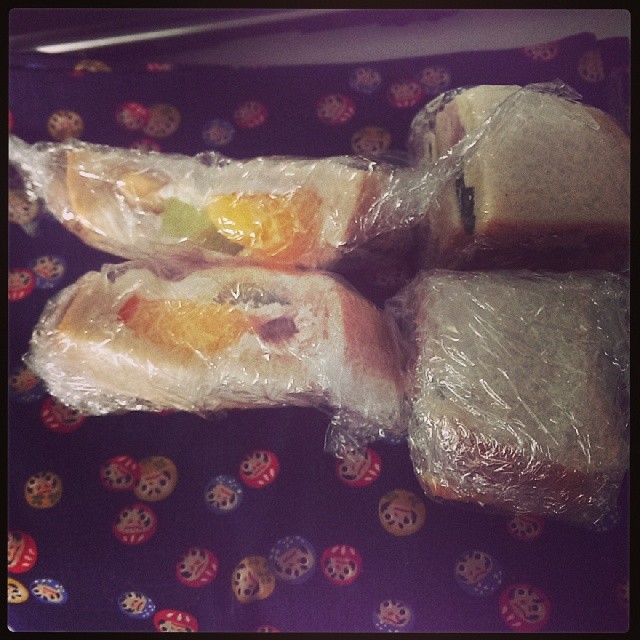This is an indoor, close-up color photograph of food items wrapped in clear plastic saran wrap, appearing to be part of someone's lunch. On the left side of the image, there are two pieces of bread that seem to have fruits on top, possibly indicating slices of a fruitcake. These fruits look like orange and green grape pieces. On the right side, there are two halves of a sandwich wrapped in saran wrap. The bread on these sandwiches appears to be rye and it's not toasted. The sandwiches on the right may contain sliced turkey, cheese, or possibly meat and vegetables.

The background features a dark blue or black cloth with a pattern of red, yellow, and blue circles. Some circles appear to have abstract faces or spots within them. The upper and lower portions of the image are slightly dark, and the photograph is notably blurry, with no printed text or words visible. The setting seems to be atop a folded tablecloth or a similar surface, with hints of a silvery or shiny object placed at the top edge of the image.